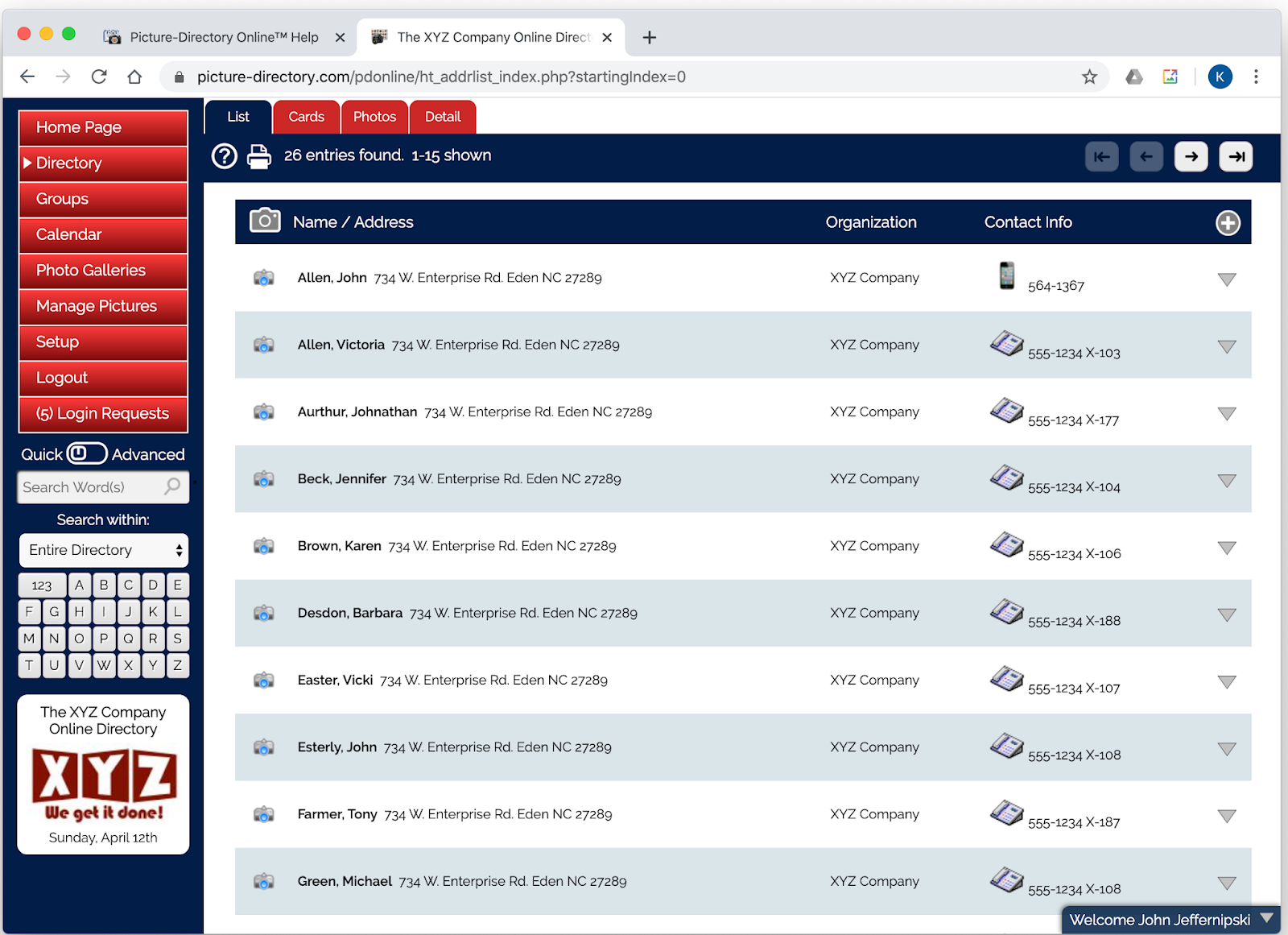Screenshot of the XYZ Company Online Directory webpage features a gray header with three circles on the left: red, yellow, and green, symbolizing typical browser window buttons, and labeled "Picture Directory Online Help." To the right, there's an "X" for closing the window, and the active tab reads "XYZ Company Online Directory."

Beneath the header, the page has a cohesive gray background. Directly below the header resides a prominent white banner bar featuring navigation icons: a left arrow, a right arrow, a refresh button, and a home button, followed by a light gray address bar that displays a populated URL.

On the left sidebar, exhibited on a navy blue background, are drop-down menus with red tabs and white text. The menu items include “Home,” “Homepage,” “Directory,” with an arrow beside "Directory," “Groups,” “Calendar,” “Photo Galleries,” “Manage Pictures,” “Setup,” “Logout,” and “Logon Requests.” Underneath, the sidebar continues with "Quick Advance," a search bar labeled “Search Words” accompanied by a magnifying glass icon, and a further option to “Search Within Entire Directory.”

The main content area begins with a white background header proclaiming "The XYZ Company Online Directory," and is highlighted in red blocks stating "XYZ: We Get It Done" alongside a timestamp "Saturday or Sunday, April 12th."

The primary section of the webpage presents an organized list in a table format, introduced by a blue tab indicating "26 entries found, 1 to 15 shown." The table columns are labeled "Name" and "Address," where names are formatted with the last name first followed by a comma and the first name. At the top of the table, additional red tabs are labeled “Cards,” “Photos,” and “Details,” offering further interactive options.